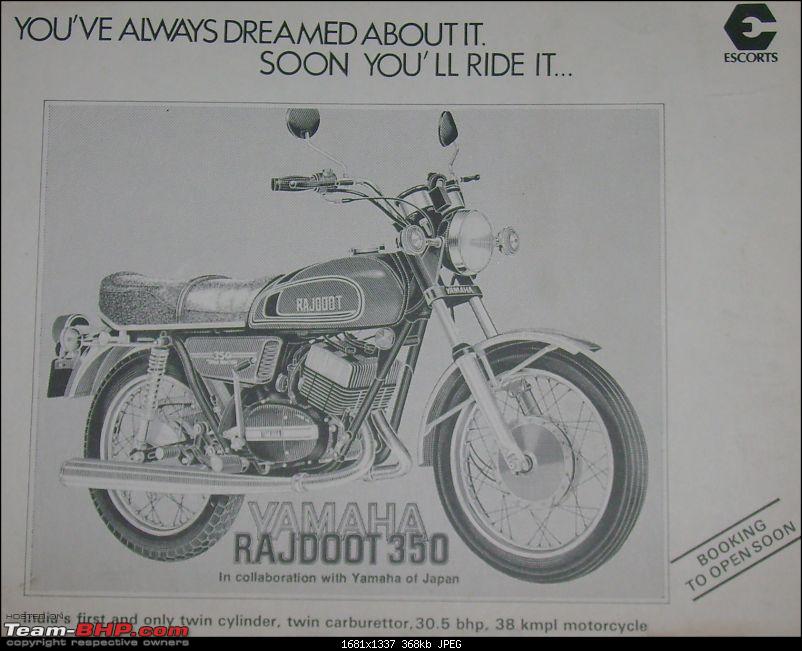This is a black and white advertisement for the Yamaha RAJ-D00T-350 motorcycle, indicating it's an older promotional piece. The headline up top reads, "You've always dreamed about it, soon you'll ride it." The image prominently features the Yamaha RAJ-D00T-350, a traditional-looking model reflecting its era. Noted for being India's first and only twin-cylinder, twin-carburetor motorcycle, it boasts specifications such as 30.5 BHP and 38 KMPL. The collaboration between Yamaha of Japan is highlighted, and the advertisement mentions sponsorship or affiliation with Escorts. In the bottom right corner, it states, "Booking to open soon." This photograph, likely sourced online, serves as a historical glimpse into Yamaha’s earlier marketing campaigns.